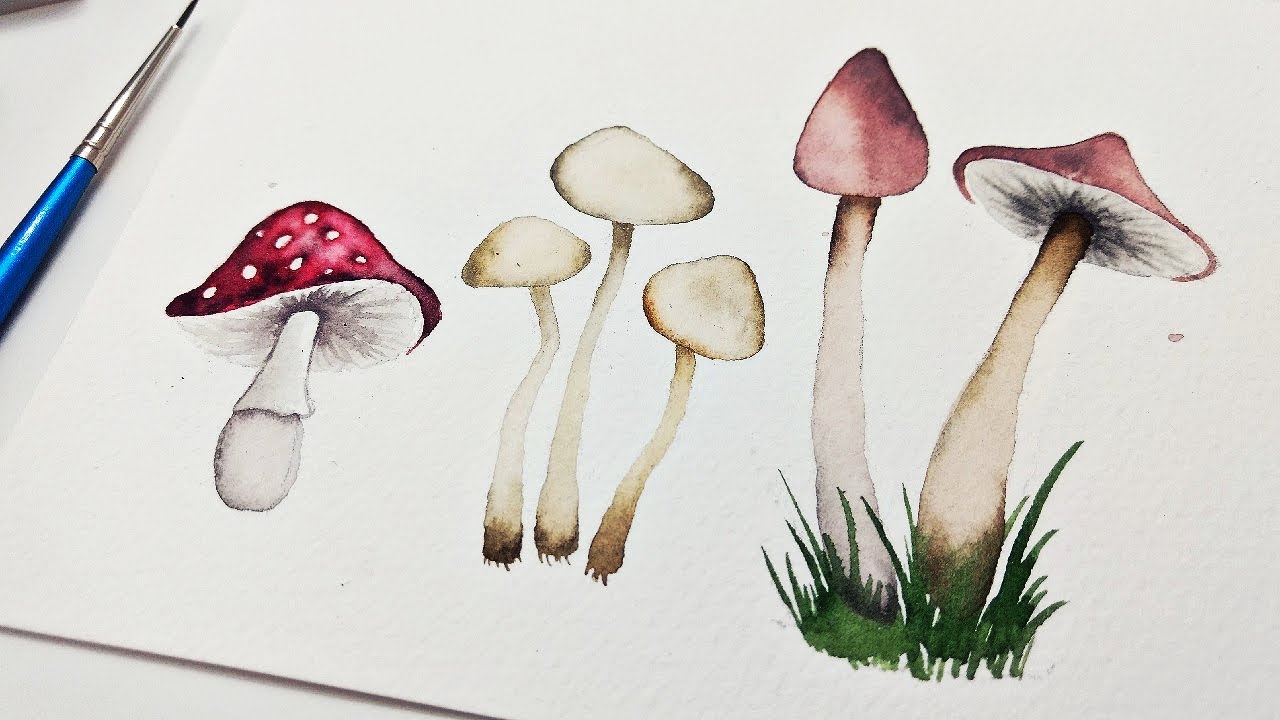This is an image of a watercolor painting positioned on an artist's drawing board. The white canvas features a detailed depiction of three types of mushrooms. In the upper left corner of the table surface, there is a blue-handled, fine-tipped paintbrush lying next to the painting. 

The painting begins on the left with a single mushroom characterized by a striking red cap adorned with white spots, reminiscent of the classic toadstool. The middle section showcases a cluster of three mushrooms, each with long white stems and subdued tan caps, suggesting a species that commonly appears after rainfall. Lastly, on the right side of the canvas, a pair of mushrooms emerges from blades of green grass. These have white stems and maroon caps, with a gradient that darkens to nearly black at the top. The canvas itself is stark white, providing a harmonious background that accentuates the vibrant details of the mushrooms.